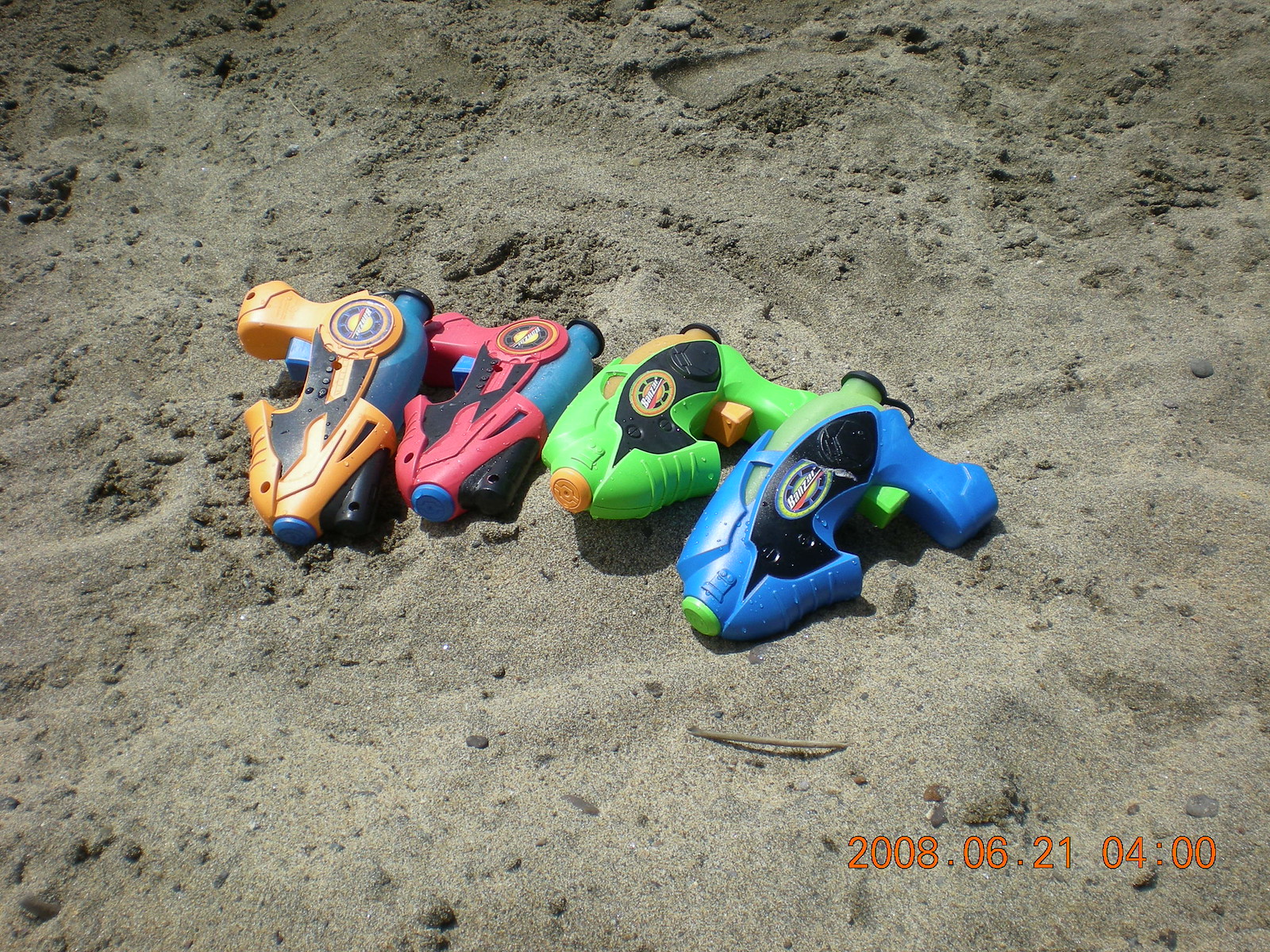This color photograph, taken on June 21st, 2008, around 4:00 PM, depicts a beach scene with four brightly colored children's water pistols lying on grayish beach sand that also contains some sticks, twigs, and stones. The sand appears to be smoothed over in certain areas, possibly to erase footprints. The water pistols, sporting a futuristic design, are arranged with their muzzles pointing downward. These approximately one-foot-long water guns include a blue one with a green tip and handle, a green one with an orange tip and handle, a red one with a blue tip and handle, and an orange one also with a blue tip and handle. Some of the guns feature black accents, adding to their vibrant appearance. All four water pistols lie side by side, creating a visually compelling scene that captures a playful summer moment.